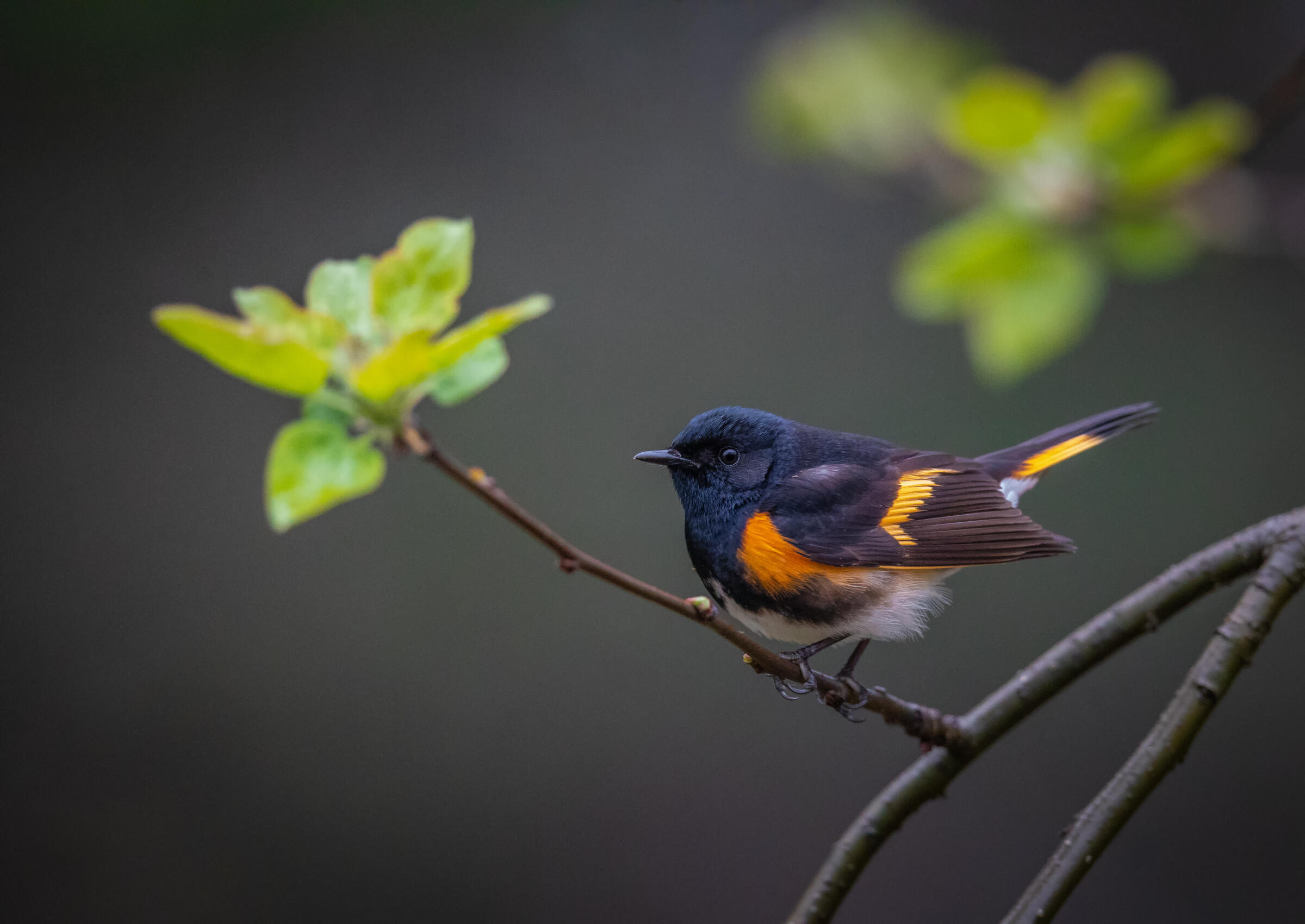This professionally shot, square, full-color photograph captures the beauty of nature with a small, vibrant songbird as its centerpiece. The outdoor image, likely taken during daylight using natural lighting, presents a detailed side profile of the bird perched on a twig adorned with green leaves. The background is primarily gray, darker at the corners, and brighter in the center, with out-of-focus green leaves and branches adding depth to the scene.

The bird, gazing to the left, displays striking colors: its head is blue, it has black eyes and a tiny black beak. The head and breast are marked with black, and its wing starts a vivid blue, transitions to gold, then brown, with a bright orange stripe. The belly is pristine white, and the tail feathers are blue and golden, with an orange streak adorning the back part. The bird's small size, approximately three to five inches long, and its elegant stance make it a mesmerizing focal point against the subtly contrasted background. The vivid hues of black, brown, blue, orange, and white, along with the green leaves, create a harmonious yet lively composition.